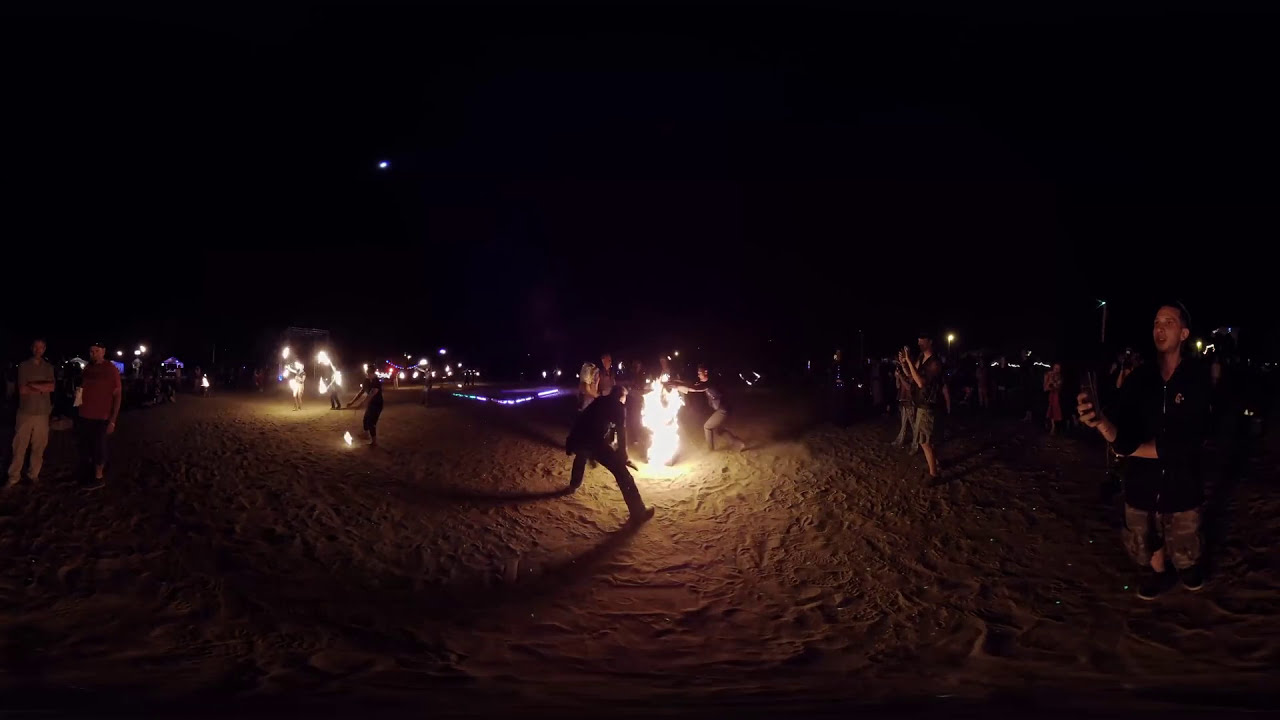In this nighttime beach festival scene, set against a dark sky with a single visible star, multiple groups of people are engaged in various activities on the sandy terrain. Centered in the image is a small bonfire that draws the attention of several individuals. To the left, a couple of people stand gazing towards the camera, with distant lights and other festival-goers faintly visible behind them. The fire, which appears to be tended by a person with their arms forward, illuminates these nearby figures. To the right of the bonfire, a person is crouched, seemingly inspecting the flames, while another person stands very close to the fire, appearing to reach into it.

In the background, faint, colorful glows, possibly purple and blue electric lights, add to the festive atmosphere. Additionally, there seem to be fire jugglers whose performances contribute to the lighting. On the far right, a person with a dark jacket holds up a cell phone, possibly to capture the event in photos or videos. Surrounding this scene, other festival-goers, including a man in a red t-shirt and another in a gray or green shirt with khaki pants, mill about, further contributing to the lively atmosphere of what might be a festival akin to Burning Man, characterized by its sandy, open environment and nocturnal revelry.